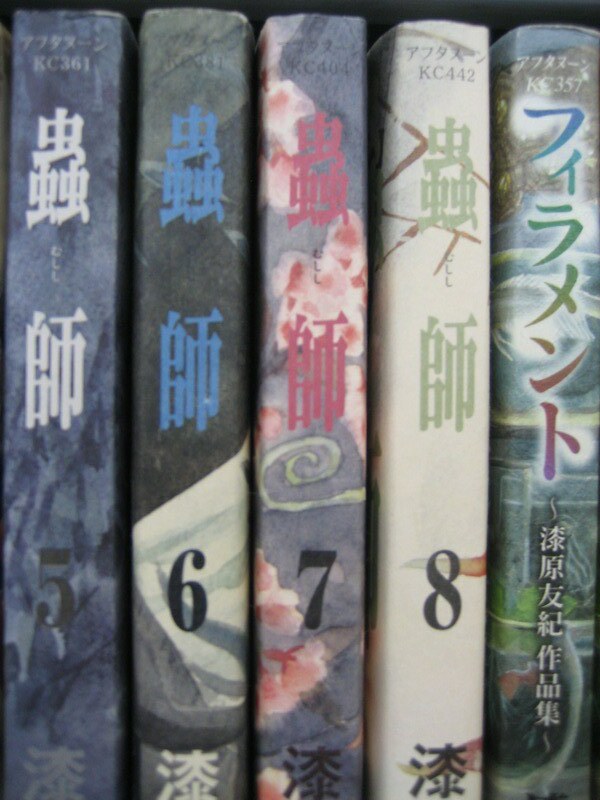This photograph captures the spines of five vertically aligned books, each showcasing vibrant and diverse covers in a foreign language, possibly Japanese. The first four books, each labeled 5, 6, 7, and 8, appear to belong to a series by the same author, as indicated by the consistent kanji characters on their spines. Book 5 sports a dark cover with light grey detailing, while Book 6 features the author's name in blue on a black background, alongside a white element that resembles a shirt collar or shoulder. Book 7 has a grey spine adorned with sunset-colored clouds and a swirl, with the author’s name prominently displayed in red. Book 8 is predominantly white with green lettering and a twig design extending onto the spine. The fifth book, distinct in its appearance, showcases different characters and an industrial image wrapping around the spine. All books are uniform in size and fill the entire frame of the photograph.